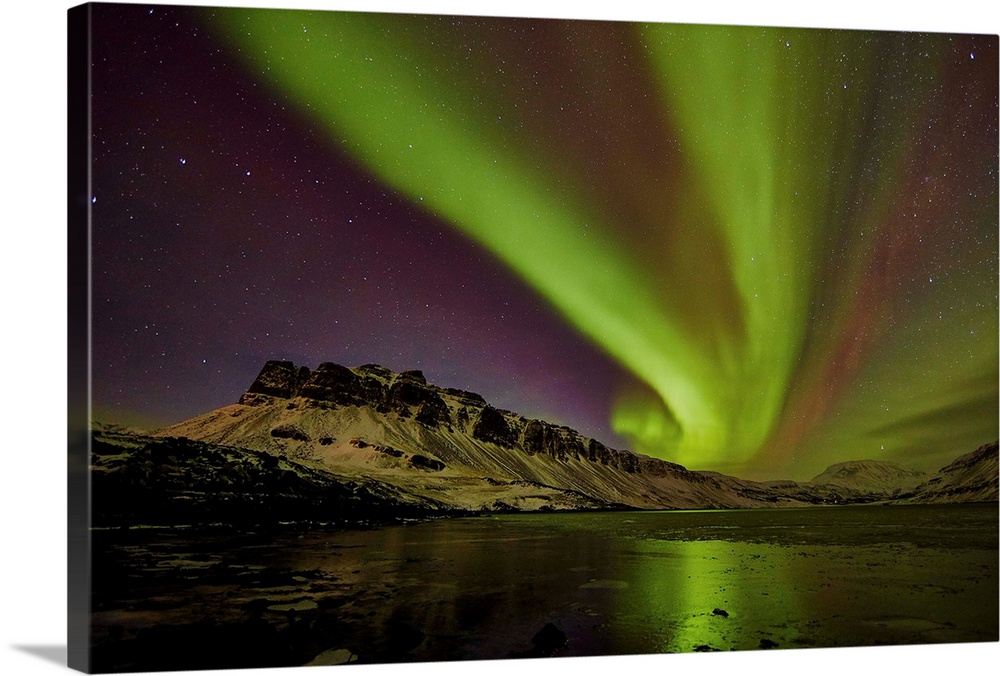A superimposed image on a tilted canvas, showing a nighttime scene dominated by a breathtaking display of the Northern Lights. The sky is a deep purple filled with stars, with a striking streak of green and hints of red aurora stretching from the foreground towards the background, primarily on the right side. A formidable rock formation mountain, colored in brown and black, runs down the center of the image and tapers off into the distance towards the right. Below the mountain, a tranquil lake reflects the mesmerizing night sky. The lower part of the image reveals a shiny lake bed, possibly dried-up, adding texture to the scene. The entire image has a slightly surreal quality, with the colors and atmosphere blending in varying degrees of intensity. The canvas casts a subtle shadow behind it, enhancing the overall depth and richness of the visual experience.